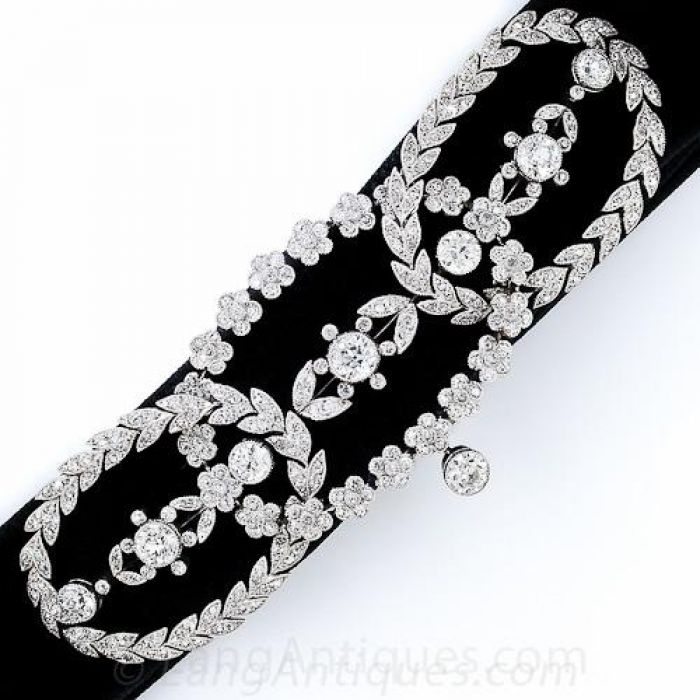The image showcases a luxurious jewelry display set against a pristine white background. Dominating the scene is a sleek black felt armature, angling diagonally from the upper right to the lower left, designed specifically to exhibit jewelry. Adorning this black structure are three exquisite diamond necklaces, each meticulously arranged to span the length of the felt arm. The central necklace stands out with a large, dazzling pendant flanked by intricate floral designs crafted from smaller diamonds, forming detailed patterns that resemble leaves and flowers. This central diamond pendant is encircled by six smaller diamonds, adding to its grandeur. The other two necklaces also feature elaborate diamond configurations, contributing to an overall presentation that sparkles with refined elegance and intricate craftsmanship.